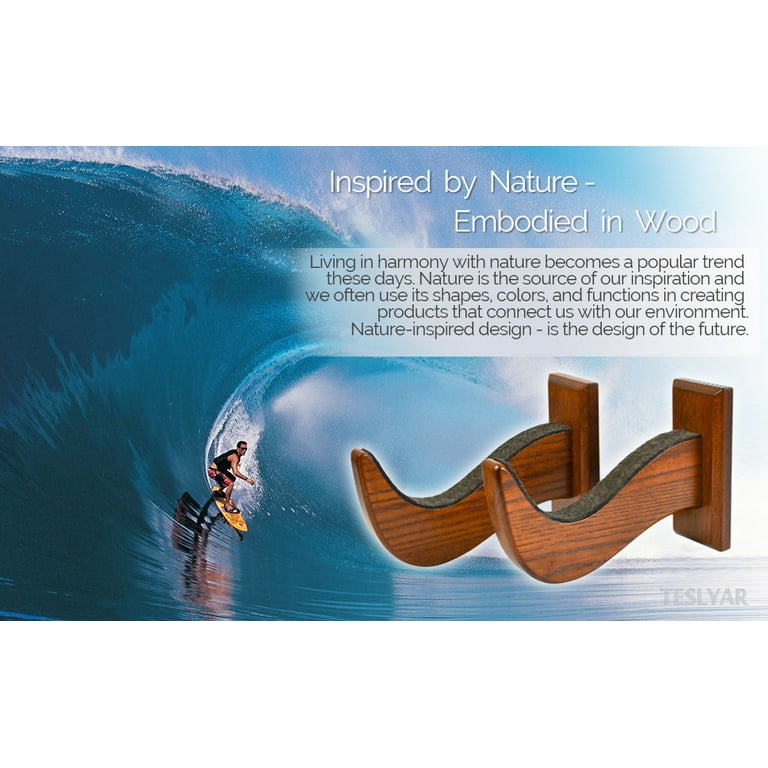This digital advertisement poster showcases a surfboard holder, featuring two wooden hooks mounted on rectangular wooden backplates, designed to attach to a wall. Dominating the advertisement is a dynamic photograph of a surfer navigating a massive green wave, with a clear blue sky in the background. The surfer, crouched with his right foot forward, rides a yellow surfboard while wearing a black life jacket and black sunglasses. 

At the top of the poster, white sans-serif text reads, "Inspired by nature, embodied in wood." Beneath it, black sans-serif text on a white panel emphasizes a growing trend: "Living in harmony with nature becomes a popular trend these days. Nature is the source of our inspiration. We often use its shapes, colors, and functions in creating products that connect us with our environment. Nature-inspired design is the design of the future."

The design of the wooden hooks subtly mimics the curves of ocean waves, reinforcing the nature-focused aesthetic promoted by the brand, TESLYAR, which is marked in a watermark in the bottom right corner of the image.